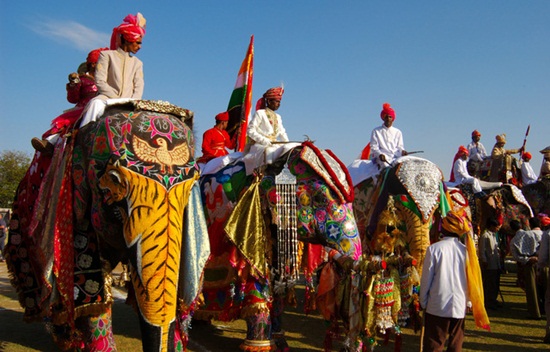The photograph captures a vibrant outdoor scene featuring a line of ornately decorated domestic elephants, adorned from head to toe in colorful cloths and intricate designs. The elephants are ridden by Indian men, all appearing to be dressed in white jackets and pants, topped with red turbans. The foremost elephant has a trunk adorned with yellow and tiger stripes, and a detailed white bird with outstretched wings on its head, complemented by a purple star featuring the number 18, hinting at a race or a ceremonial event. Each elephant displays its unique vivid decorations in hues of blue, red, yellow, and orange. Some of the elephants also feature Indian flags and other embellishments. The ground beneath them is dirt, and the sky above is a clear blue with a scattering of white clouds, enhancing the vibrancy and festivity of the scene. On the ground in front, more men are gathered, contributing to the lively atmosphere of this striking and colorful tableau.